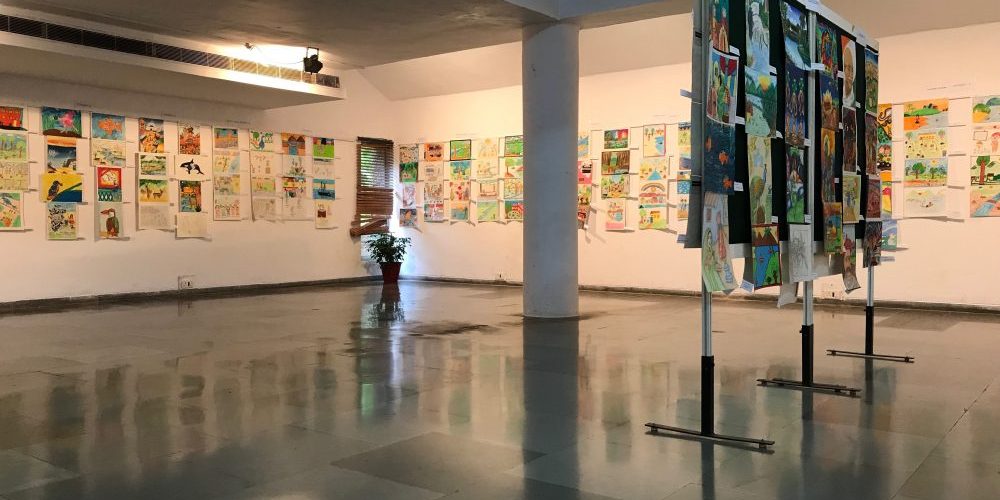This image depicts a large, open room that appears to be inside an art museum. The walls are a crisp white, while the floor is covered in gray tiles, some of which vary in shade without forming a discernible pattern. Dominating the center of the room is a substantial column that reaches up to the ceiling, reinforcing the spaciousness of the area. 

In the far corner, a window with brown blinds allows natural light to seep in, complemented by a potted plant sitting beneath it. Artworks adorn the walls, arranged neatly in rows and columns with four pieces in each column, wrapping around the entire room. These pieces are vibrant and colorful, potentially the works of children, featuring a variety of subjects, although specific details are hard to make out.

A spotlight is suspended from the ceiling, illuminating the displayed artwork. Additionally, there is a display stand on the right side of the room, also showcasing several pieces of artwork, adding to the gallery-like atmosphere of the space.